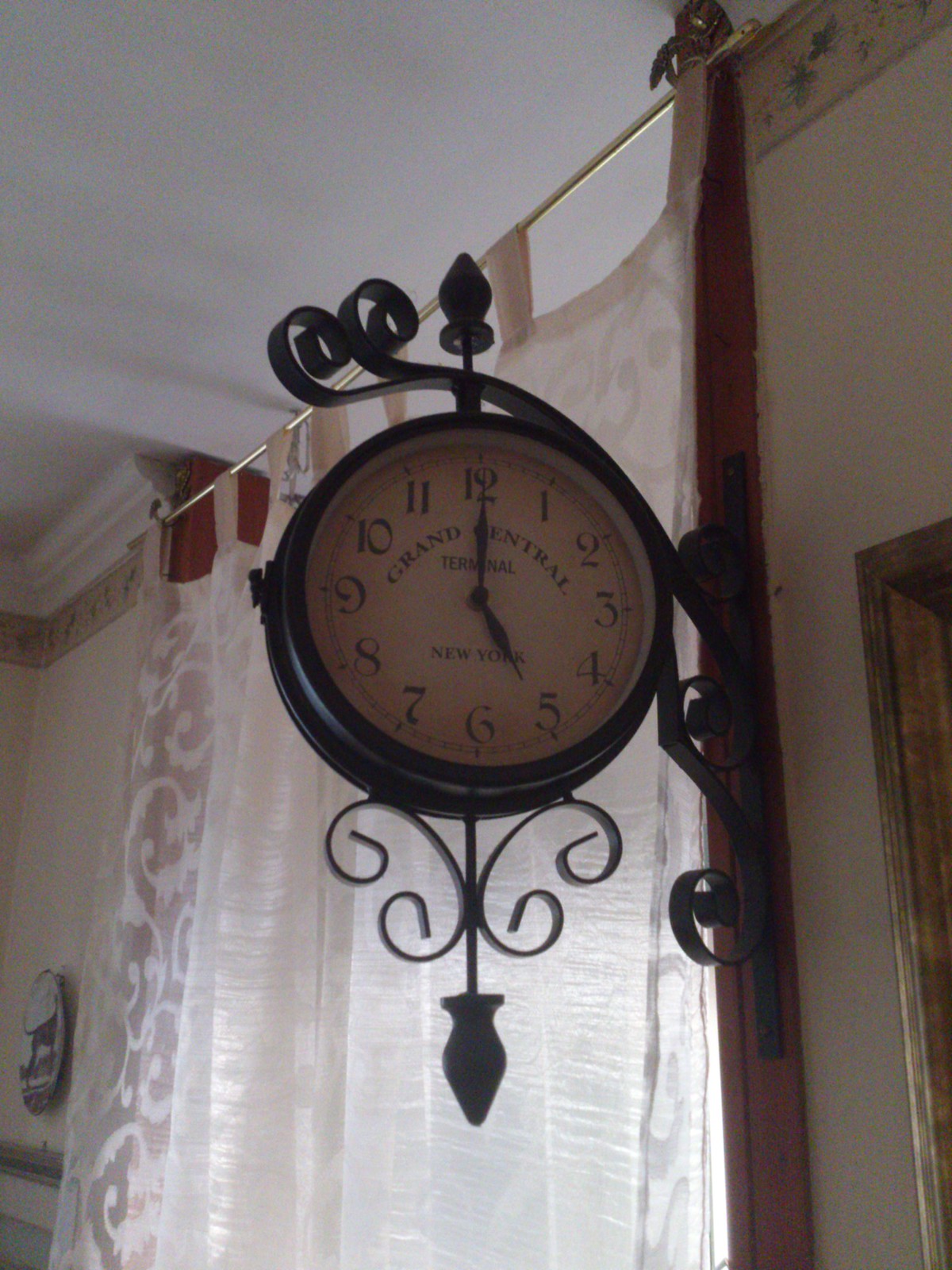The image captures the interior of an old home reminiscent of a grandmother's house, centered around an antique-style clock that evokes the design of those found in train stations. The clock, which indicates the time as 5 o'clock, features a black frame with intricate, swirly metal designs on the top and bottom, reminiscent of backward apostrophes. It reads "Grand Central Terminal, New York," suggesting it holds an antique charm. The clock is unique in that it projects from the wall sideways, like a traffic sign, rather than sitting flat.

Behind the clock, light pink curtains with a gold-like cord suggest a window or a doorway divider. The wall itself appears to be covered in wallpaper with a combination of pink and brown hues. Just visible on one side of the wall is a painting of a standing dog, while on the other side, a decorative plate can be seen. The overall photograph gives a sense of nostalgia, enriched by the traditional decor and muted color palette, possibly enhanced by a vintage filter effect.